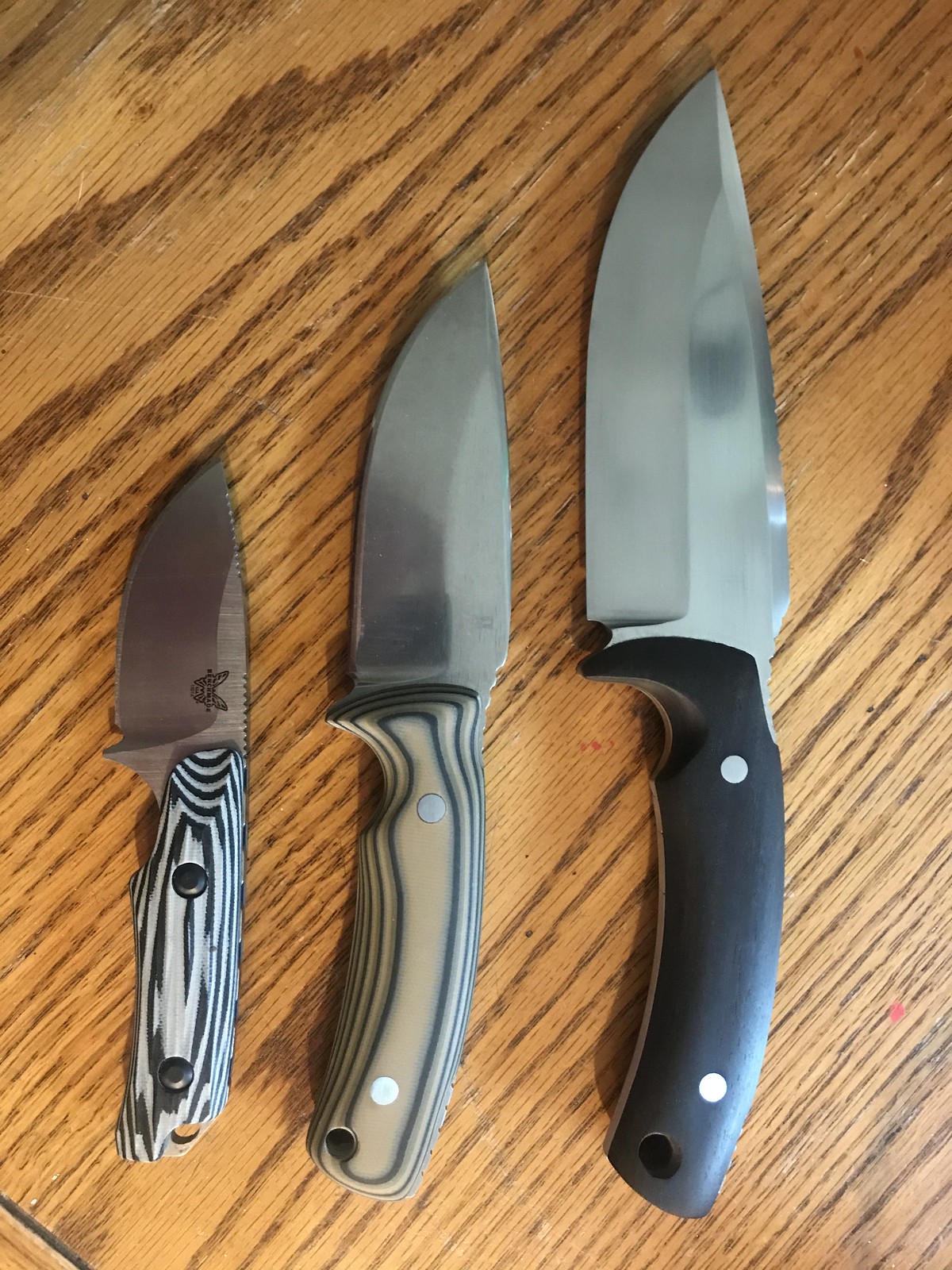This is a high-quality, portrait-style photograph of three knives arranged side by side on a wooden table, showcasing a gradual increase in size from left to right. The background features a wood finish with darker, noticeable strokes of brown. Each knife boasts a silver, non-serrated, stainless steel blade. The handles are each unique in design: the smallest knife on the left has a zebra print handle; the middle knife sports a khaki version of the zebra print; and the largest knife on the right has a solid black handle. Notably, all the handles are equipped with two silver dots, presumably functioning as rivets securing the blade to the handle. The blades face left and lie flat against the table, providing a stark contrast to the rustic wooden surface.